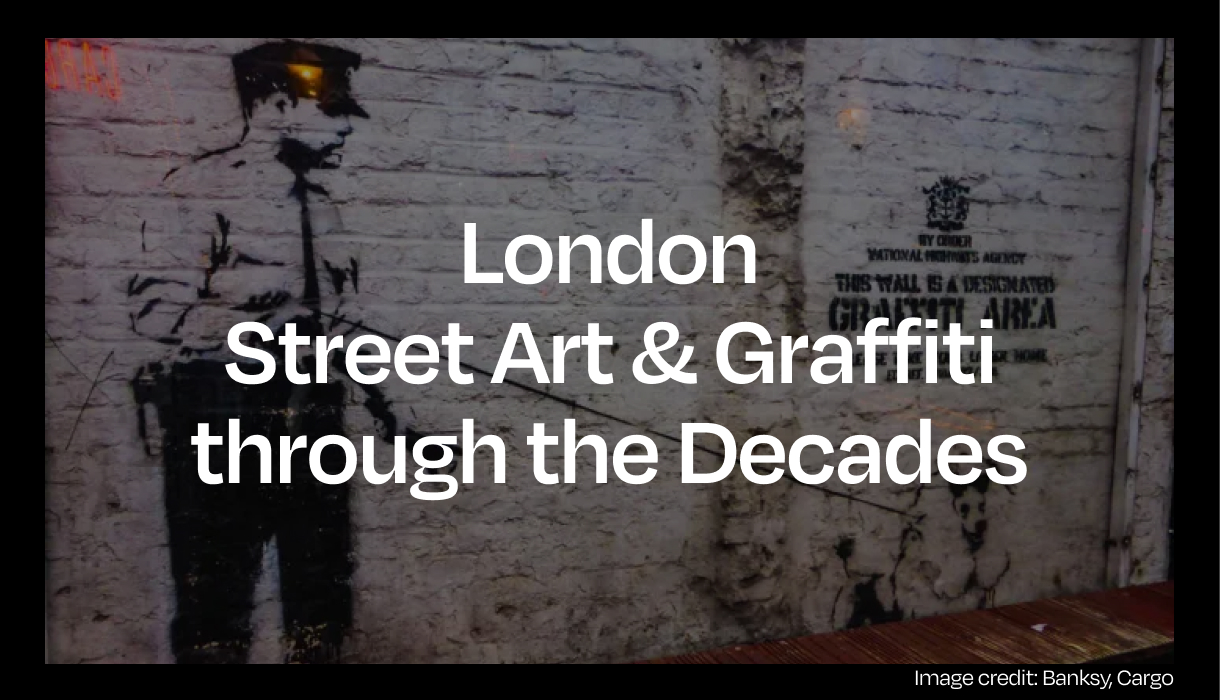The image features a white-painted brick wall adorned with a stencil or spray-painted black outline of a police officer. The officer, positioned on the left side, is depicted wearing a cap, a white shirt, a tie, and dark pants, with various equipment on his belt. The scene is framed with a thin black border. Bold white text across the center of the image reads, "London Street Art and Graffiti Through the Decades." At the bottom right, there is an image credit that states, "Image credit: Banksy, cargo." Additionally, black spray paint on the right side of the wall designates it as a "graffiti area," indicating a legally permissible space for graffiti.